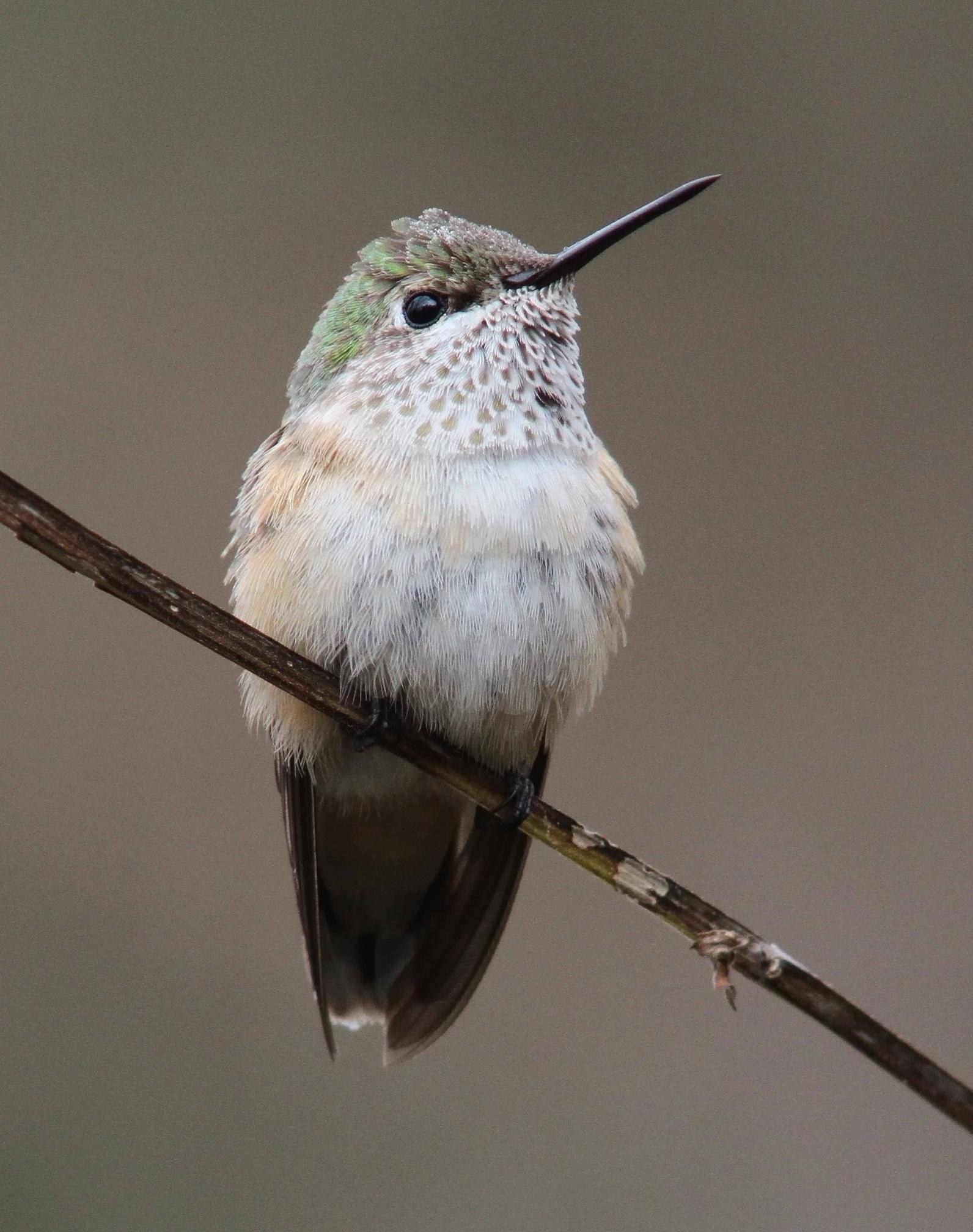This image features a close-up of a small songbird, possibly a hummingbird, perched diagonally on a slender, dark brown twig against a tan to grayish-brown background that gradates subtly from green at the top to rust in the middle and green again at the lower left. The bird is centered in the frame, facing the camera with its head tilted to the left, and its long, slender, and pointy black beak is directed towards the upper right corner of the image. The bird has black eyes and a cap of muted, varying shades of green with a gray patch down the center. It has a white face with brown speckled spots, a white chest, and light brown feathers on its wings. The bird's tail is a dark grayish-brown color, though it appears shadowed. The bird's black feet are wrapped securely around the twig, adding to the overall delicate and intricate detail captured in the photograph.